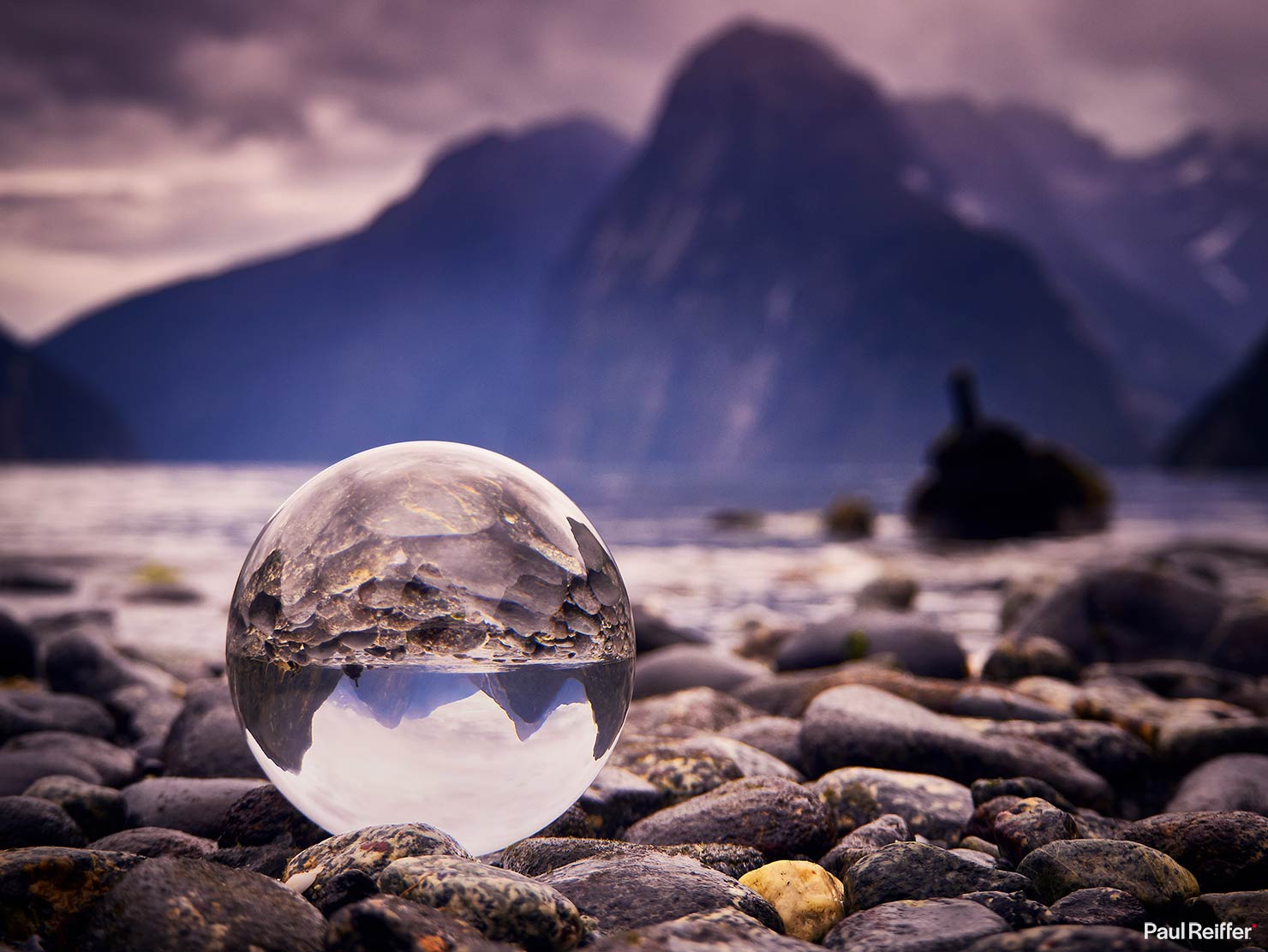The image, taken by photographer Paul Reifer as indicated by his name in white writing at the bottom right corner, showcases a serene outdoor scene at dusk. Dominating the foreground is a spherical, glass-like object acting as a reflective globe, portraying the surroundings in an inverted manner. Nestled among smooth, dark gray rocks worn by water, the globe reflects the scattered stones and a lone standout yellow pebble. Behind these rocks lies a tranquil body of water, likely a lake, extending into the distance where imposing, jagged mountains rise sharply. These mountains, tinted with shades of dark gray and purple, are set against a heavily clouded sky painted in hues of light purple and gray, with no direct sunlight visible. The composition beautifully captures the contrasting elements of the reflective globe, the earthy rocks, the serene lake, and the dramatic mountainous landscape under a moody sky.